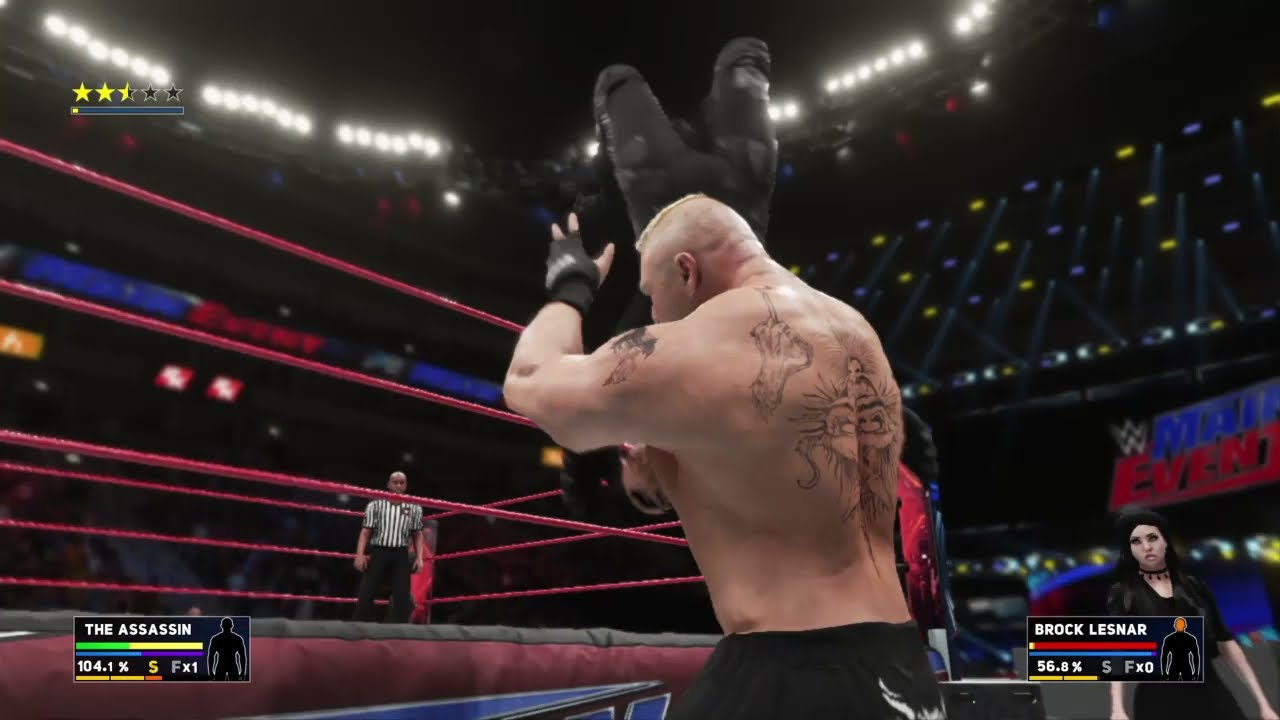The image is a highly detailed screenshot from a WWE wrestling video game featuring Brock Lesnar. Brock, a big, muscular man with a shaved head and a bit of blonde hair on top, is outside the ring on the left side. He is wearing black shorts and fingerless gloves, showcasing his distinctive back and arm tattoos. He is in the middle of suplexing an opponent, who is flipped upside down with his legs bent behind him like a scorpion. The opponent is light-skinned with dark eyeliner and is clad in black military-looking stretch pants. 

In the background, a digital stadium full of seats and glaring lights can be seen. Inside the ring, marked by its red ropes and red ring skirt with a blue logo, stands a thin, bald black referee, attentively watching the action. To the right of the screen, a black-haired woman wearing a choker, black shirt, and hood is visible.

Interface elements of the video game frame the scene: the top left corner displays a horizontal row of five stars, with 2.5 stars yellow and the rest black, beneath a blue bar with a touch of yellow at the far left end. The bottom of the image features health status boxes—“The Assassin” on the left, representing Brock's opponent, and “Brock Lesnar” on the right, presumably with red indicating Brock's health status.